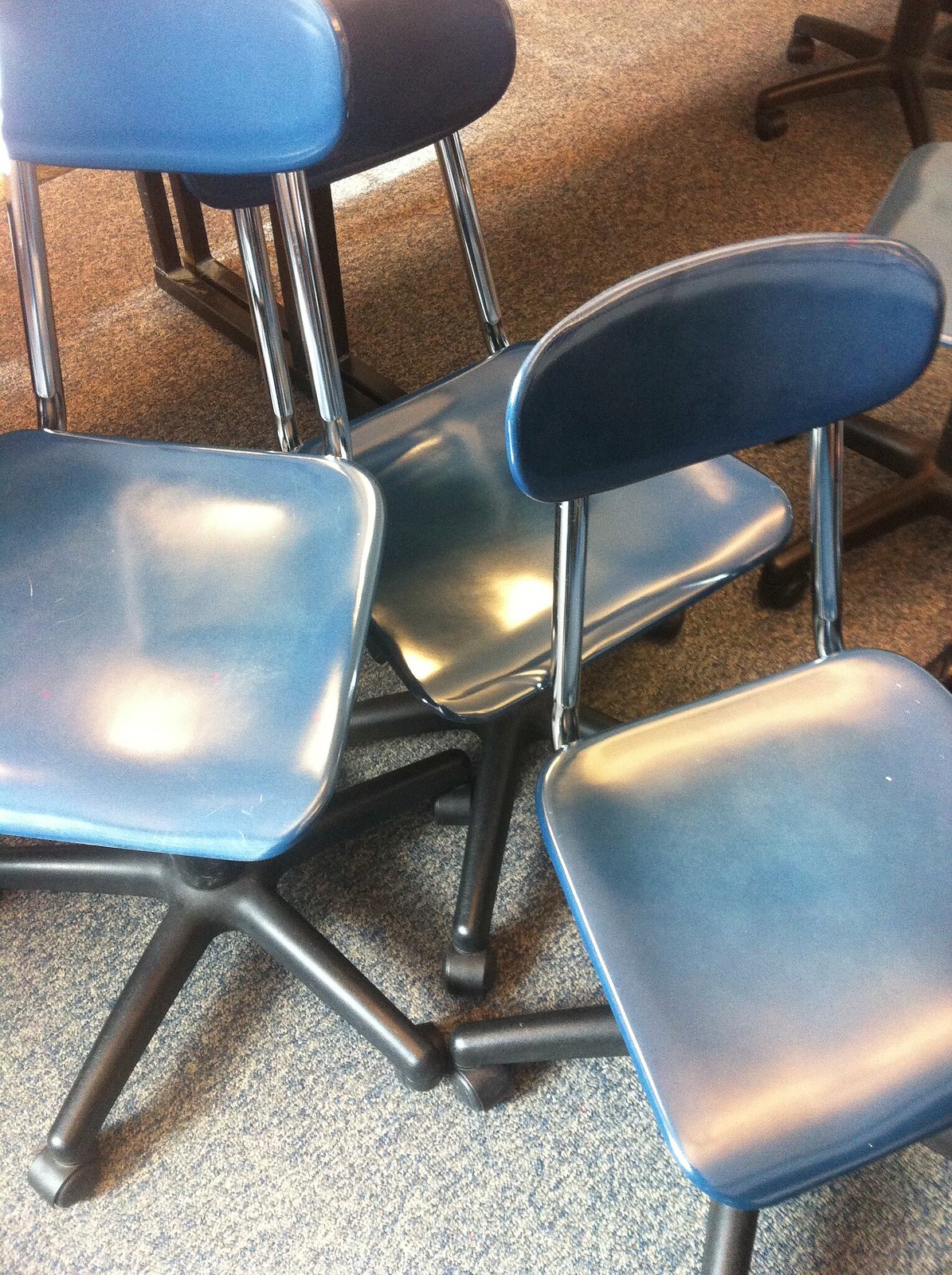This image depicts a grouping of blue office chairs with unpadded, small, oval-shaped backs mounted to the seats via two chrome metal rods. The seats are flat, and the bases of the chairs consist of five-legged star patterns equipped with black wheels. The chairs catch the reflection of classroom lights, adding a silvery, shiny appearance. The setting includes a white floor with black spots, and there is no presence of desks—only more of the same type of chairs scattered throughout the background. The photograph is taken from a slightly top-down angle, revealing additional chairs partially visible among the central cluster.